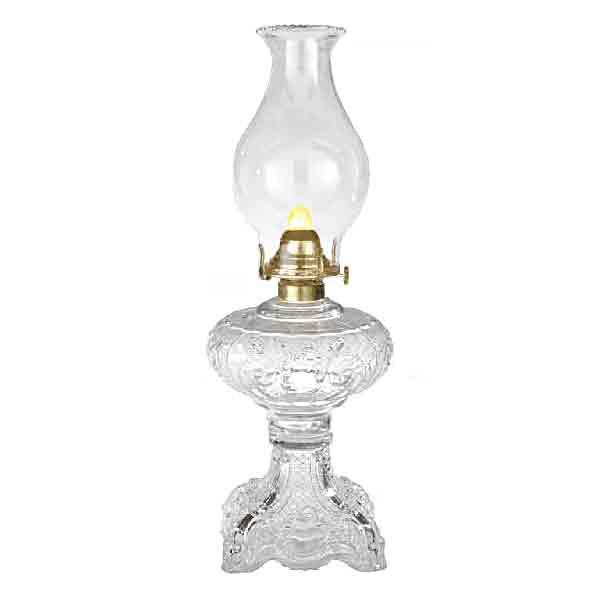This photo features an exquisite antique crystal oil lamp, potentially dating back to the late 1800s or early 1900s. Standing approximately 18 to 19 inches tall, the lamp showcases intricate and ornate Victorian-style detailing. The base is made of textured cut crystal, adorned with delicate patterns and embellishments that enhance its vintage charm. The bowl portion, where oil is stored, is clear and elegantly designed. The burner, situated above the bowl, is a silverish-gold fixture that supports a simulated yellow flame. Atop the lamp is a traditional clear glass hurricane globe, reflecting the classic design of early kerosene lamps. Set against a stark white background, this beautifully crafted lamp stands alone, its historical allure and craftsmanship vividly highlighted.